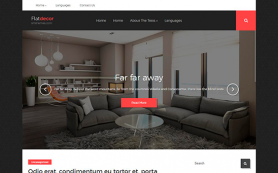This screenshot captures a web page, predominantly featuring an image of a modern living room. The image is quite small and not easily readable due to its zoomed-out nature. In the image, a contemporary styled living room is adorned with medium gray furniture, centered on a gray mauve rug. A circular coffee table with a glass top occupies the middle of the room. The living room is illuminated by large floor-to-ceiling windows fitted with retractable shades, allowing natural light to fill the space. In the back corner of the room, bookcases and pendant lights add to the room’s sophisticated ambiance. The walls are painted a muted mauve tan, enhancing the modern aesthetic. The web page itself has a sleek design with a black outline accented by red highlights. At the bottom of the page, framed by a white border, the word "condominium" is visible. Superimposed on the living room image, the phrase "Far Far Away" is prominently displayed, though the smaller text beneath it remains unreadable due to pixelation.